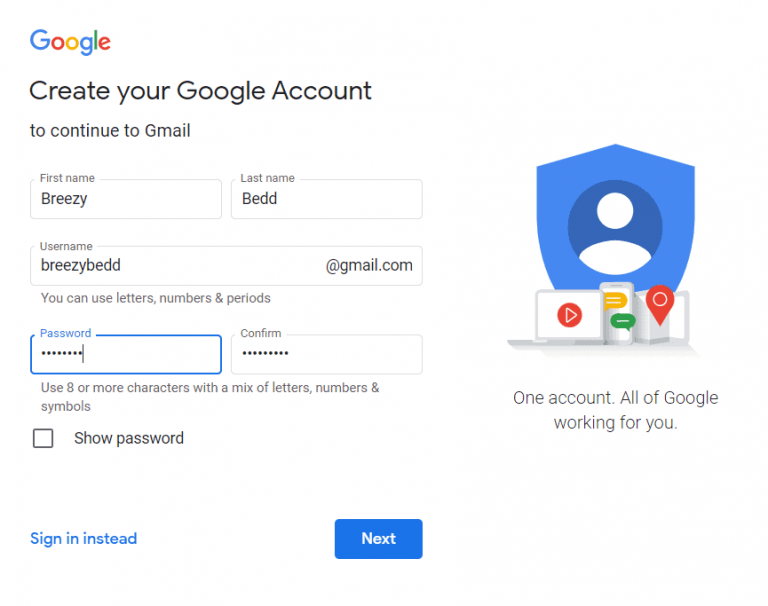A detailed screenshot depicting the process of creating a new Google account is shown. At the top, the familiar "Google" logo is prominently displayed. Below it, the text "Create your Google Account" appears, directing users to continue to Gmail. The form fields request personal details, starting with "First name" entered as "Breezy" and "Last name" as "Bed." For the "Username" field, the user has input "breezybed@gmail.com."

Under the username field, a note indicates that users can include letters, numbers, and periods. Further down, two password fields are visible, both containing obscured, starred-out characters to protect privacy. Instructions below these fields emphasize using eight or more characters, combining letters, numbers, and symbols. An unchecked option to reveal the password is present.

Additional text encourages users to "Sign in instead" or click "Next" to continue. At the bottom, Google's branding slogan, "One account. All of Google working for you," reinforces the unified nature of their services. This screenshot captures a typical step in setting up a new Gmail account.